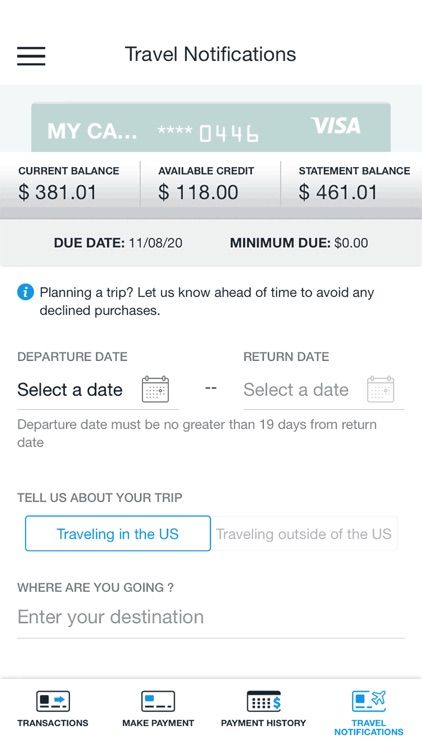The image depicts a segment of a credit card statement or user interface related to a credit card account. 

At the top of the image, there is a white header featuring three black dashes aligned on the left side. Centrally positioned, the words "Travel Notice" are displayed. Below this header, a section with a greenish-gray background includes text in white that reads "MyCA..." Followed by this text, there are four stars and the number "0446." Towards the right side of this section, the Visa logo is prominently displayed.

Beneath this header, there is a statement summary presented in gray and black. It shows the following details: "Current Balance: $381.10," "Available Credits: $118," and "Statement Balance: $461.01," indicating the user's current financial status. A note specifies that the due date for the payment was 11-08-20 and that the minimum payment due was $0, implying that it has already been settled.

Following this, there is a helpful reminder in white text: "Planning a Trip? Let Us Know Ahead of Time to Avoid Any New Client Purchases." Under this message, the section outlines fields for inputting travel details. The label "Departure Date" appears in gray, with an instruction in black underneath that reads "Select a Date with a Calendar." On the right-hand side, the label "Return Date" is also in gray, accompanied by the instruction to "Select a Date." Additional text clarifies that the "Departure Date must be no greater than 19 days from the Return Date," although the phrasing seems slightly confusing.

A section titled "Tell Us About Your Trip" is highlighted in blue, offering two options: "Traveling in the U.S." (highlighted) and "Traveling Outside the U.S." (grayed out). It prompts users to enter their destinations.

At the bottom of the image, there are navigation options labeled "Transactions," "Make a Payment," and "Payment History." The link for "Travel Notifications" is highlighted in blue.